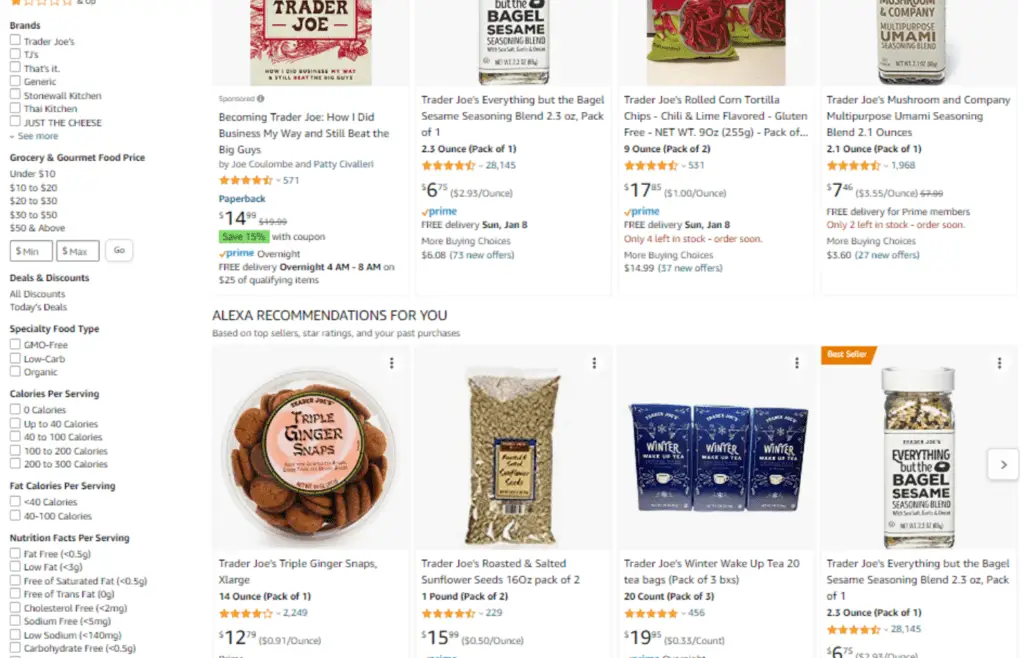The image is a screenshot of search results on Amazon.com, displayed in a horizontal landscape format with a white background. 

On the left-hand side, there is a vertical column featuring various filters to refine the search results. 

At the top of this column, under the "Brands" category, there are options such as:
- Trader Joe's
- TJ's
- That's It
- Generic
- Stonewall Kitchen
- Thai Kitchen
- Just the Cheese
- Seymour
- Grocery and Gourmet Food

Under "Price," there are selections such as:
- Under $10
- $10 to $20
- $20 to $30
- $30 to $50
- $50 and above
Along with two boxes for entering a minimum and maximum price, accompanied by a "Go" button.

Further down, under "Deals and Discounts," options include:
- All Discounts
- Today's Deals

The "Specialty Food Type" category includes filters for:
- GMO-free
- Low-carb
- Organic

"Calories Per Serving" can be adjusted with:
- Zero to 40 calories
- 40 to 100 calories
- 100 to 200 calories
- 200 to 300 calories

"Fat Calories Per Serving" features:
- Less than 40 calories
- 40 to 100 calories

"Nutritional Facts Per Serving" offers:
- Fat-free (0.5g)
- Low-fat (less than 3g)
- Free of saturated fat (less than 0.5g)
- Free of trans fat (0g)
- Cholesterol-free (less than 2mg)
- Sodium-free (less than 5mg)
- Low-sodium (less than 140mg)
- Carbohydrate-free (less than 0.5g)

Displayed product results include:
- Trader Joe's Everything But The Bagel Sesame Seasoning Blend
- Trader Joe's Rolled Corn Tortilla Chips

These products prominently feature items from Trader Joe's.

This detailed layout of filters and product listings highlights the variety and specificity of search options available on Amazon.com, particularly for Trader Joe's products.